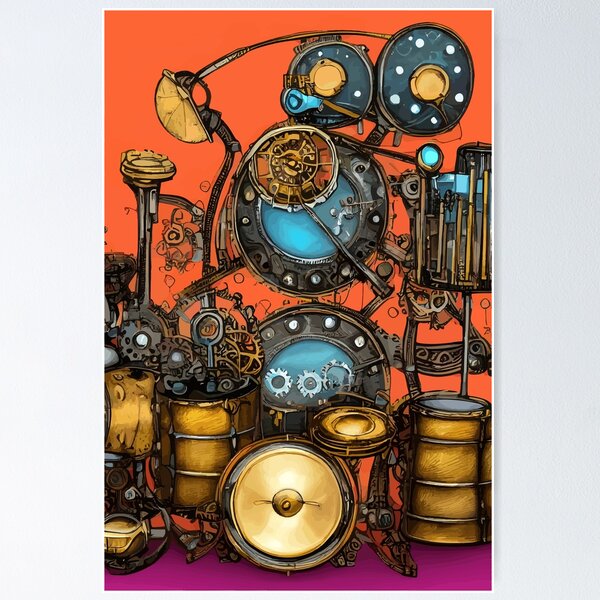The image is an intricate and ultra-modern steampunk sculpture that evokes the essence of a one-man band. Dominated by an assortment of brass, golden, and metal components, this elaborate artwork features a plethora of gears, hammers, cymbals, and tubes. Among its numerous detailed elements, there is a prominent gold barrel that resembles a drum, situated alongside another gold-colored metal piece which also looks drum-like, and a large circular object with a gold center reminiscent of a bass drum.

In the forefront lies an assortment of additional metal pieces, including two ship windows stacked vertically at the back, and what appear to be black speakers. The lower portion of the sculpture is an assembly that suggests a steampunk version of a cymbal combined with a bass drum, complete with wheels, pulleys, discs, and axles. The entire assembly exudes a noisy and mechanized feeling, as if it could spring to life in a cacophony of sound at any moment.

The background is a striking red, while the floor is adorned with a lavender hue, adding to the surreal and vivid nature of the scene. Every inch of this automated one-man band overflows with the industrial aesthetic typical of steampunk art, meticulously combining common and obscure objects into a cohesive, visually fascinating apparatus.